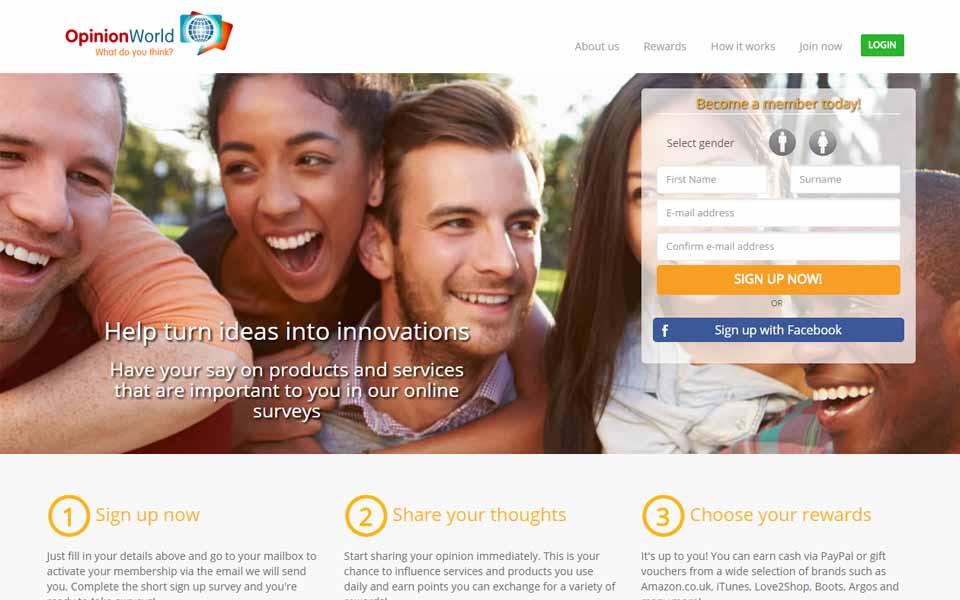The image displays the homepage of a website called "Opinion World." The website prominently features the tagline, "What do you think?" and encourages visitors to become members. The central theme of the site is to help users influence products and services through online surveys. Users are invited to join the platform to express their thoughts on various topics and, in return, earn rewards.

In the upper right-hand corner of the page, there is a navigation menu with options such as "About Us," "Rewards," "How It Works," "Join Now," and "Login." Below this, the site instructs potential members on how to sign up: they can select their gender (male or female), enter their name and email address, and then proceed by clicking "Sign Up Now." 

Further down the page, there’s an explanation of the registration process. It involves filling out the registration form, activating membership via an email that will be sent to the user’s mailbox, and completing a short sign-up survey. Once registered, members can begin sharing their opinions immediately. The platform highlights that this is an opportunity to influence the products and services used in daily life while earning points that can be exchanged for rewards.

Members can choose from a variety of rewards, including cash via PayPal or gift vouchers from popular brands such as Amazon.co.uk, iTunes, and Love2Shop. The overall message is clear: by joining Opinion World, users can make a little extra money or receive gift cards in exchange for their survey participation.